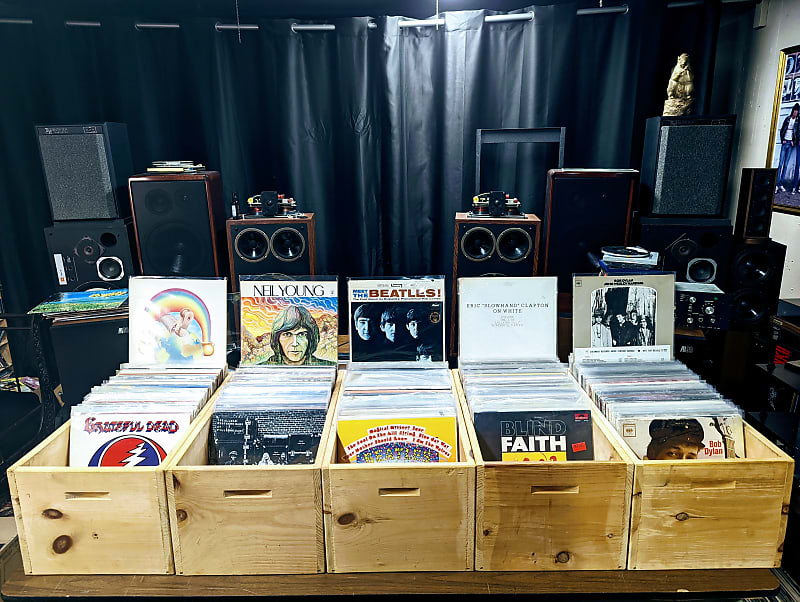The photograph captures an interior room setting dominated by a vintage musical theme. At the forefront, there is a row of five wooden boxes with metal legs, each meticulously organized with musical records. Notably, one record sticks out at the back of each box, prominently featuring artists such as the Grateful Dead—with their iconic album cover showcasing a human skull with a white lightning bolt—The Allman Brothers posing in an alleyway, as well as records from Blind Faith, Bob Dylan, Neil Young, The Beatles, and The Band. These boxes rest on a wooden table. Surrounding the wooden boxes, there is an array of audio speakers—ranging from four to six speakers per unit—some stacked and arranged in pairs, both to the left and right. A black silk curtain forms the backdrop, with posters adorning the walls. Additionally, there are a couple of chairs and another table that holds a record player and a box designed for bass and different sound outputs, adding to the room’s retro audio vibe.